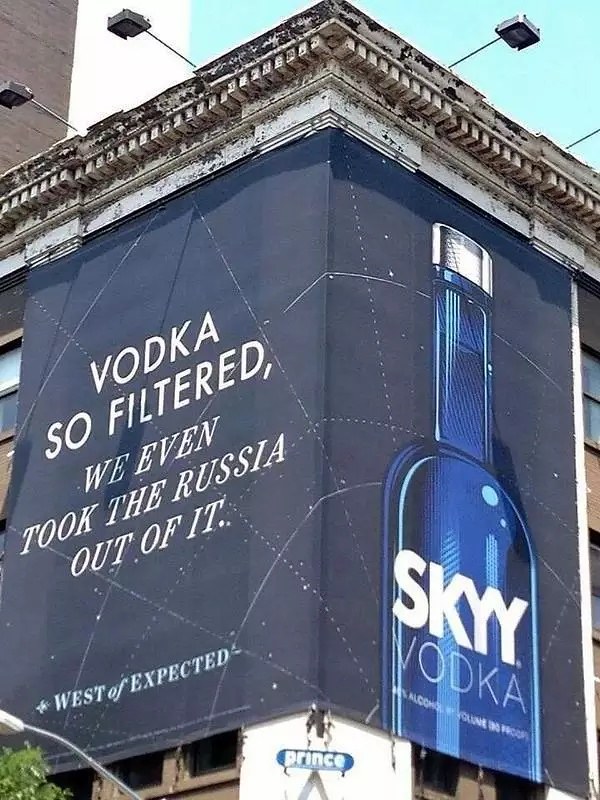The image showcases a billboard-style advertisement for Sky Vodka prominently displayed on the corner of an older cement building in a likely urban setting. The ad creatively spans across two sides of the building, appearing as if it is folded over the corner, making a striking visual impact. The deep blue advertisement features a large, white-text slogan that reads, "Vodka so filtered we even took the Russia out of it. West of expected." Directly below the text, a picture of a Sky Vodka bottle is depicted, with a deep dark blue bottle, white writing, and a silver cap. Above the corner of the building, a teal-tinged sky provides a backdrop, giving the scene an almost surreal ambiance. The building itself is adorned with a large cornice at the top, with lights overhanging, adding to its aged yet stately appearance.